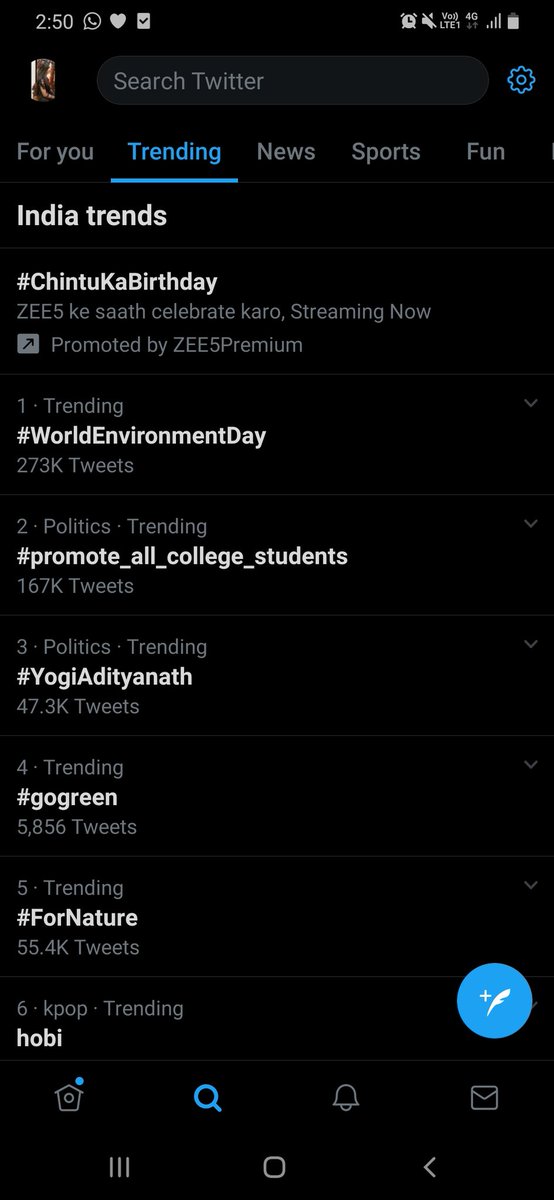**Caption:**

A screenshot from an older version of the Twitter app in dark mode, featuring a black background. The user is on the "Trending" tab, showcasing trends specific to India under the "India trends" header in the search bar. While the profile icon of the user is visible, it is not clearly discernible. 

The trending topics include:

1. **World Environment Day** - ranked as the top trend
2. **Chintu Ka Birthday** - promoted by ZEE5 Premium
3. **Yogi**
4. **#ForNature**
5. **Hobi (H-O-B-I)**

The text predominantly appears in white, with trends reflecting a mix of environmental themes and events/individuals relevant to Indian Twitter. One promoted trend, "Chintu Ka Birthday," stands out, advertised by ZEE5 Premium.